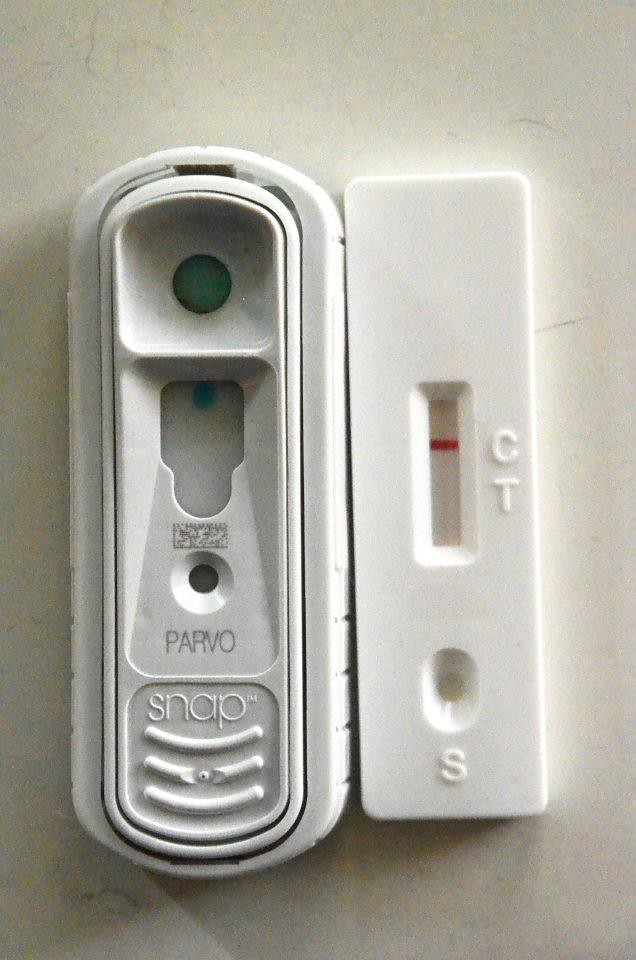The image presents a meticulously detailed close-up of what appears to be a COVID-19 test kit or a similar viral diagnostic device, photographed on a blank white surface. On the left side of the image is a white plastic apparatus with a design featuring several key components. At the top, there's a small circular window. Below this window lies an opening with a distinguishable blue dot inside. The plastic section is further enhanced with a pattern resembling a QR code, followed by another small circular opening.

Continuing downward, the word "PARVO" is prominently displayed in black letters. Adjoining this section is a bordered area with raised, wave-like structures pointing downward. At the top, above these features, the word “SNAP” is written in raised white letters.

To the right of this structure lies a long rectangular test strip, also white, centered around a screen displaying a horizontal red line. Adjacent to this screen, on the right, is the letter "C." Below the screen sits the letter "T." At the bottom of this test strip, a circular opening is marked with the letter "S." All these letters "C," "T," and "S" appear raised, much like the "SNAP" lettering on the test to the left.